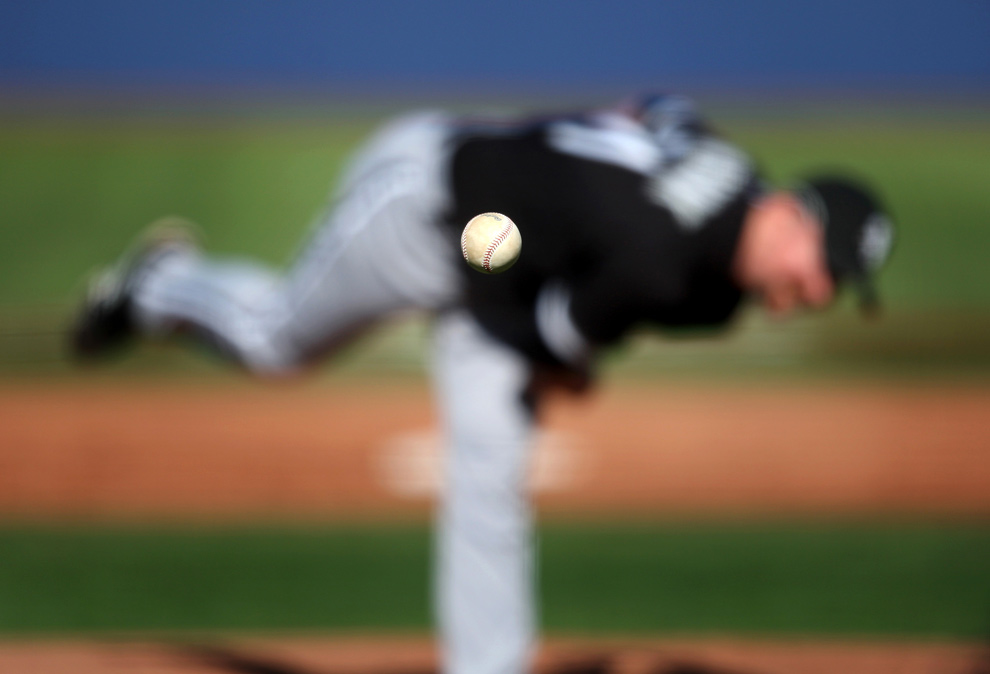A dynamic photograph captures a baseball pitcher mid-game, dressed in gray pants, a black shirt, and a matching black hat, right after releasing a pitch. The shot is taken from the perspective behind the catcher, with the camera focused precisely on the baseball, rendering the background slightly out of focus. This creates an intriguing effect where the ball appears to be floating crisply in the center of the frame. In the slightly blurred background, the field, second base, outfield, and boundary wall are visible, hinting at the expansive surroundings. It's a bright, sunny day, as evidenced by the distinct shadow of the pitcher on the mound, his right leg raised high in the air. The baseball itself shows signs of wear, with a noticeable dirty spot on its underside, adding to the authenticity and intensity of the moment captured.